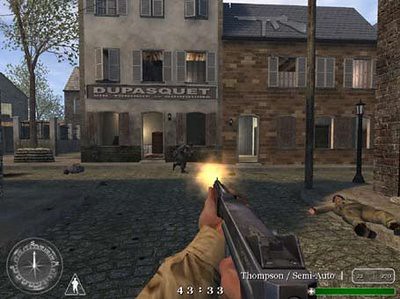A screen capture from a World War II-era video game showcases an intense battle on a cobblestone street in an old European town. From the first-person perspective of the main character, the player grips a Thompson semi-automatic machine gun, evident from the muzzle flash as the weapon is fired. A compass in the bottom left corner provides navigational orientation, while the game's timer in the bottom right indicates that 43 minutes and 33 seconds remain. The focal point of the image features a soldier in a gray uniform who appears to be the target of the protagonist's gunfire. Nearby, another character lies motionless on the street, presumably a casualty of the ongoing conflict. The detailed setting and action-packed scene evoke the tumultuous atmosphere of wartime Europe.